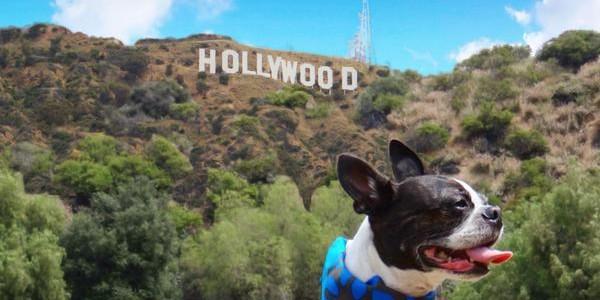This is a photo of a black and white Boston Terrier dog, prominently superimposed against the iconic Hollywood sign that is positioned on the Hollywood hills. The Hollywood sign features its characteristic white lettering, and the hills appear dry with green and brown patches of shrubbery, indicative of an arid climate. The dog has pointy ears, dark eyes and nose, and is looking slightly to the side with his mouth open, tongue sticking out as if panting. He is wearing a blue jacket, visible up to the collar, as the rest of his body is cropped out of the frame, which itself is formatted in a four by three ratio. Above the Hollywood hills, the sky is adorned with white puffy clouds, and there is a utility pole visible on the hill. The image quality is somewhat low, with only the dog slightly more in focus than the background.